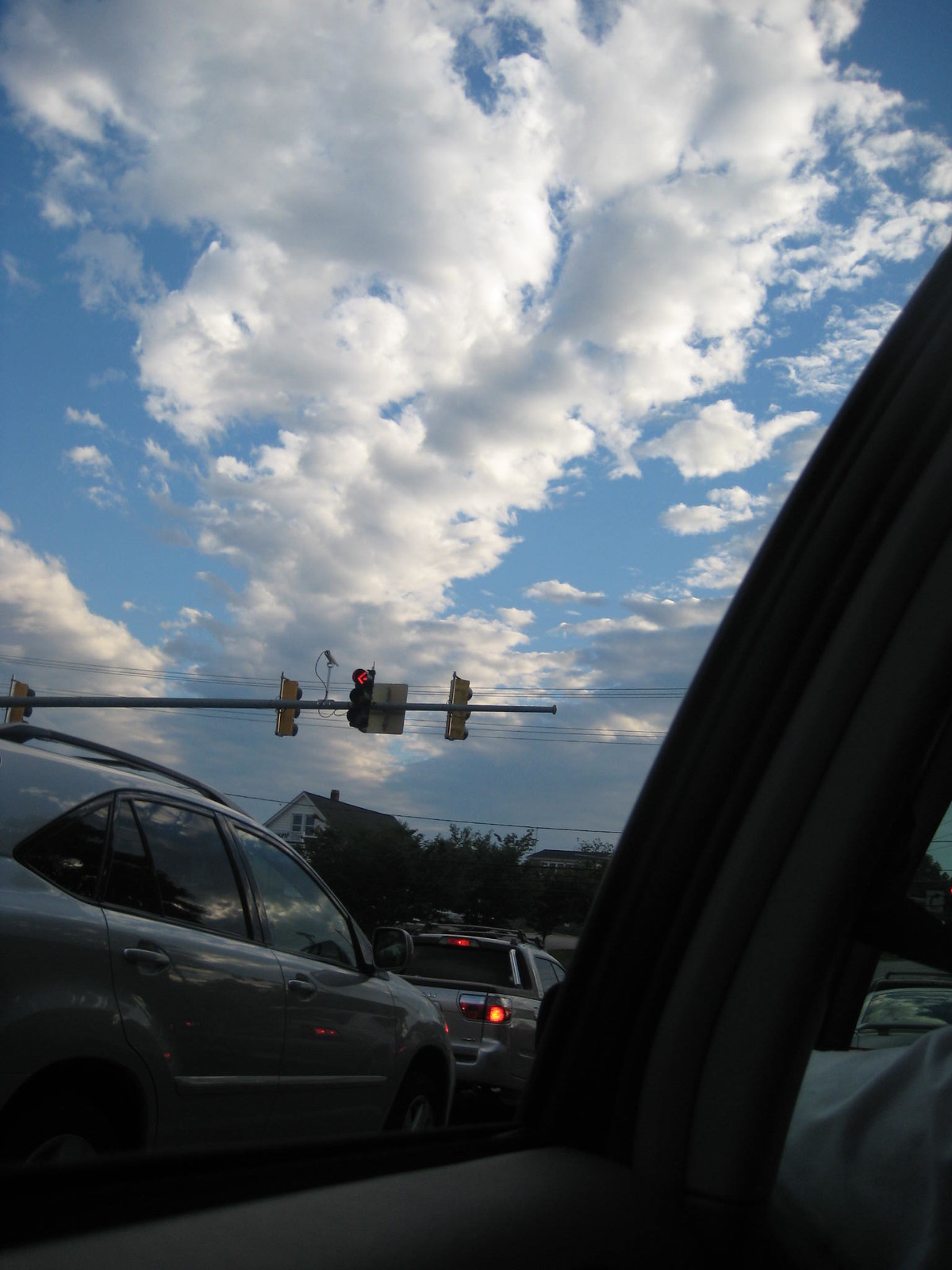A view from the back passenger side window reveals a scenic outdoors and part of the car's interior. The focus is on the sky with its blue expanse dominated by large, puffy clouds that extend across the center of the frame. To the left, two vehicles are stopped at a traffic light; a smaller white truck in front and a silver SUV with tinted windows behind it. Looming above them is a large horizontal pole with three traffic lights: one facing the traffic and two facing the opposite direction. A traffic light camera is perched above, angled down towards the intersection. In the bottom left corner, the tan interior of the car door is visible. On the bottom right, part of the driver’s arm, clad in a white shirt, enters the frame. This detailed scene captures a moment in transit with elements of both the vehicle and the surrounding environment.